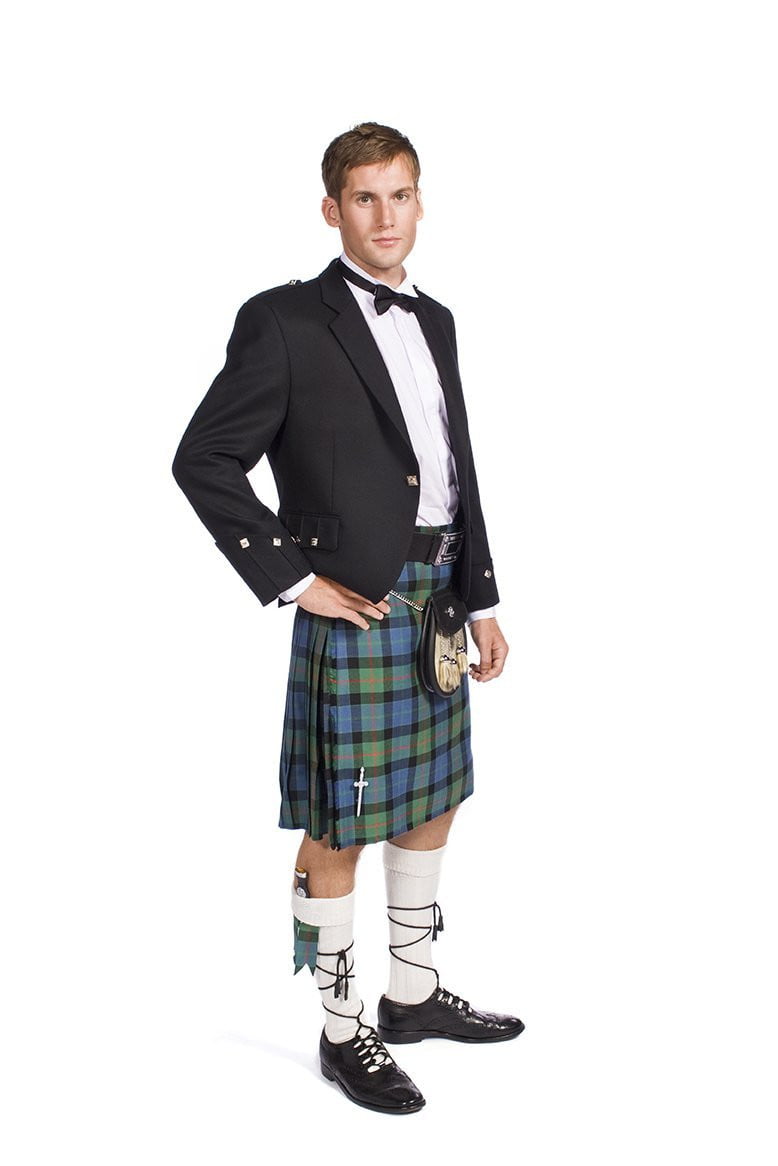The photograph appears to be professionally taken, possibly for an advertisement, set against an all-white background. It features a young white male in his 20s with short blondish-brown hair and a serious expression. He is dressed in a unique blend of formal and traditional attire. He is sporting shiny black dress shoes with intricate lace-up patterns that wrap around his calves, paired with white knee-high socks. His ensemble includes a blue, green, black, and red tartan kilt, accessorized with a leather waist pouch and a cross pin attached to the front. The kilt is secured with a black belt featuring a notable buckle. Complementing this are a crisply ironed white dress shirt and a black suit jacket, topped off with a black bow tie. The young man stands confidently with one hand on his hip and the other hanging by his side, exuding a composed and poised demeanor.